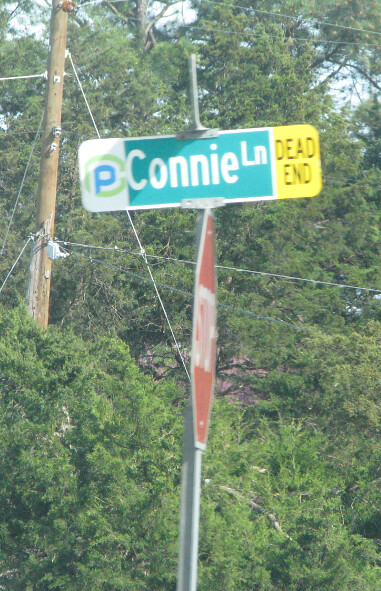This detailed photograph captures a street sign mounted on a silver post. At the top of the post, there's a stop sign, although it's angled in such a way that only the red portion is discernible. Directly below the stop sign is a green sign with white text that reads "Connie Lane." Adjacent to this, on the same sign assembly, is a yellow sign with black text indicating a "Dead End." Further to the left on the same assembly is a white sign featuring a blue "P" enclosed within a green circle. Above the stop sign is an additional, unreadable street sign. The backdrop features a dense cluster of trees and a telephone pole adorned with multiple lines.